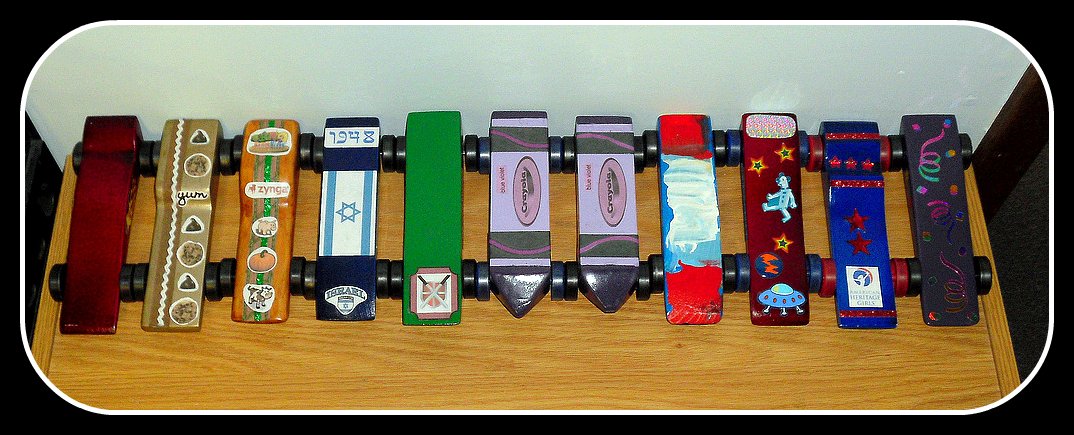This is a photograph consisting of 11 miniature wooden cars lined up along a shelf. They each exhibit a diverse range of colors and designs, with several of the cars having a narrow wedge shape and small black wheels. The cars are meticulously decorated with paint and stickers giving them unique identities: a red car, a gold one featuring chocolate chips and the word "Yum," an orange car with "Forzinga," one adorned with the Israel flag, a green car, and two purple cars marked with the Crayola logo. Notably, there's also one with a clown, a spaceship, and stars. The photograph is set within a black border with rounded edges, containing a white inner frame that highlights the horizontal arrangement of these vertical, wheeled objects on a wooden surface.